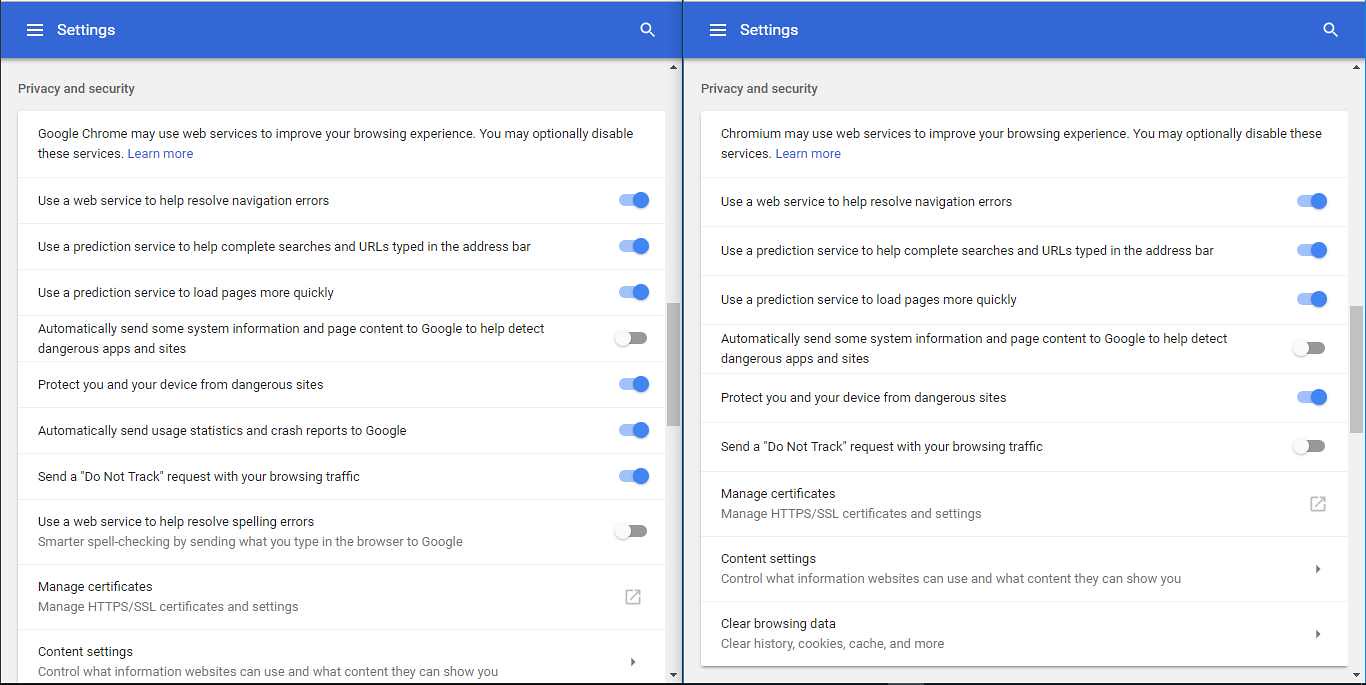In the image, we observe two side-by-side screenshots displaying the same webpage, split vertically. The right screenshot appears slightly blurrier than the left.

Starting with the left screenshot, at the very top, there is a long rectangular bar with a blue background. On the far left of this bar are three horizontal white lines, symbolizing a menu. To the right of this icon, the word "Settings" is prominently displayed. Continuing to the right end of this bar, a magnifying glass icon representing a search function is visible.

Below this top bar, the page is titled "Privacy and Security," which is clearly indicated. Directly beneath this title is a large white rectangular section containing various settings options in black text. These options detail different privacy and security features such as "Google Chrome may use web services to improve your browsing experience," "Use a web service to help resolve navigation errors," and "Protect you and your device from dangerous sites." Each option has a corresponding checkbox to its right, some of which are highlighted in blue, indicating that they are enabled, while others are grayed out, denoting they are disabled.

On the right side, the screenshot mirrors the left but with some distinct differences in the checkboxes’ statuses. Some options that are checked on the left side are unchecked on the right, and vice versa. Additionally, towards the bottom right of the right screenshot, some items such as "Manage certificates," "Content settings," and "Clear browsing data" are not accompanied by the blue check marks seen in the left screenshot.

In summary, this detailed image comparison highlights the different privacy and security settings configurations in a web browser's settings page, with varying checkbox statuses between the two sides.